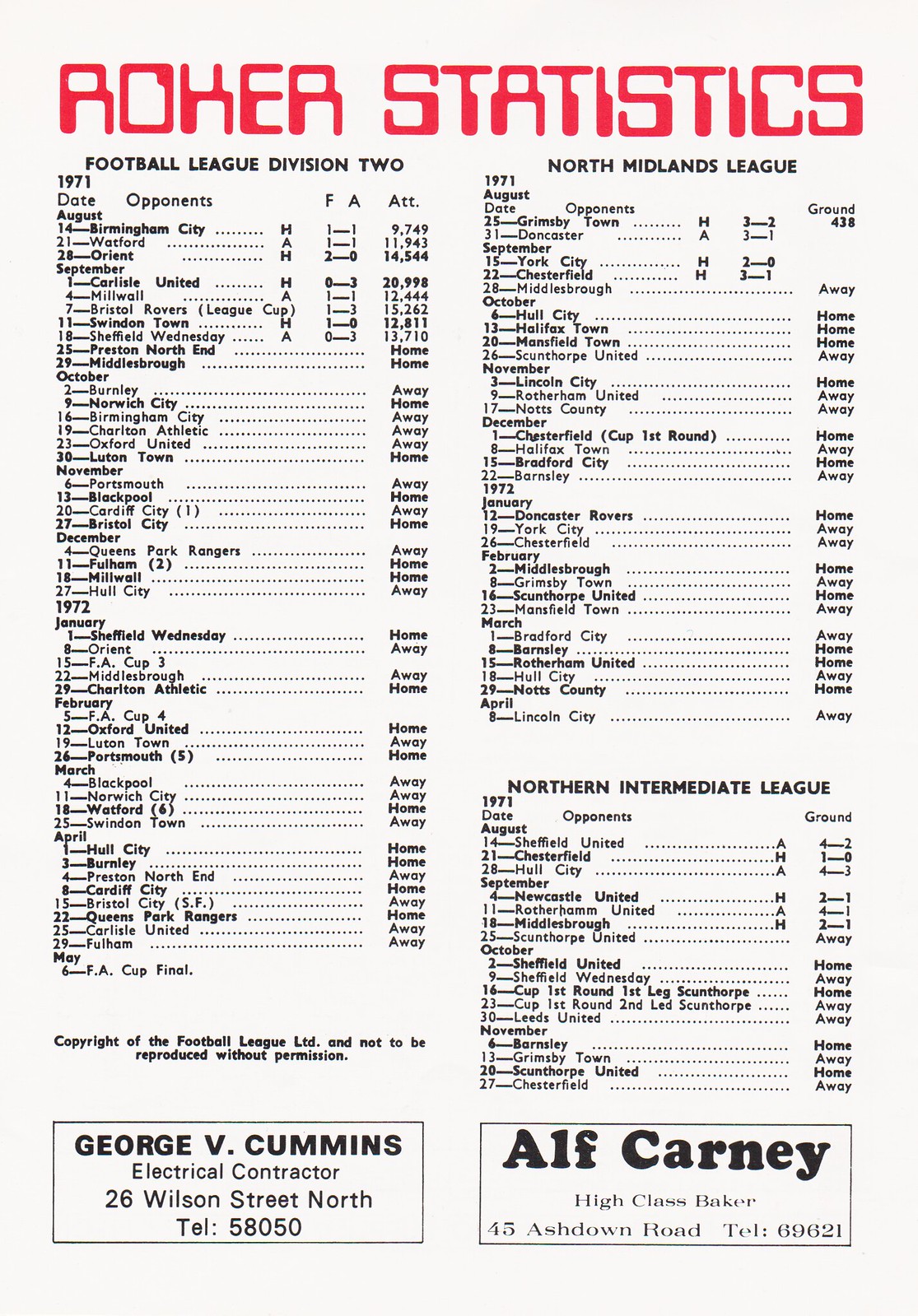This is a detailed photograph of the inside page of a football program booklet. At the top of the page, "Roker Statistics" is prominently displayed in bold, red capital letters. Below this heading, the page is split into two main sections, each containing a list of dates, opponents, records, and attendance for various matches. The left section features the heading "Football League Division II" with dates such as August 14, August 21, and August 28, 1971. The right section, although not explicitly detailed in its heading in the shared information, mirrors the left in its structure with its own list of match details. Both sections have smaller headings like "North Midlands League" and "Northern Intermediate League," emphasizing the comprehensive nature of the statistics provided.

At the very bottom of the page, two rectangular advertisements are placed side-by-side. The left advertisement is for George B. Cummins, an Electrical Contractor, located at 26 Wilson Street North, with the contact telephone number 58050. The right advertisement promotes Alf Carney, a High Class Baker, based at 45 Ashdown Road, with the contact telephone number 69621. The overall layout is set against a light grey background, with the text in black, making the red heading stand out prominently.

Overall, the image captures a thorough and organized presentation of football statistics interspersed with local business advertisements, reflective of the period's typical program design.